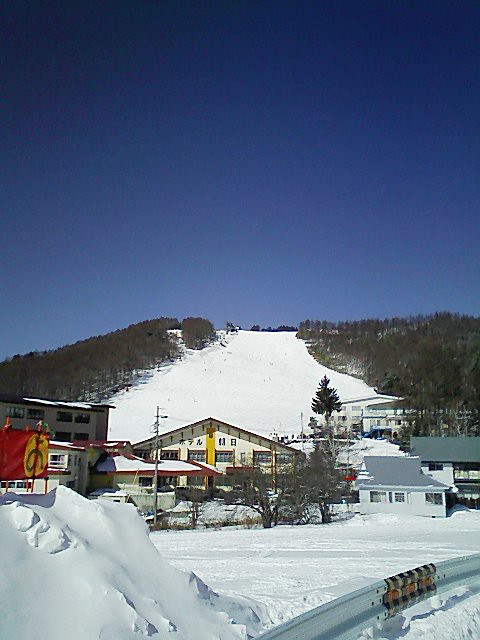This color photograph, in portrait orientation, captures a bright, sunlit day with a striking deep dark blue sky in the background. The central focus is a very tall snowy hill, not quite a mountain, with rows of dark green trees flanking either side, giving it a false appearance of a ski slope, but it's much smaller. In the foreground, dominating the lower half of the image, is a large white building with Japanese characters at the top, featuring a single dark gable and multiple windows, suggesting it might be a ski lodge. Surrounding this central building are additional structures, and at the bottom right corner, a curving steel guardrail is seen partially buried in a pile of snow. The sky transitions from a dark blue at the top to a lighter blue near the hill's summit, enhancing the overall realism and representational style of the photograph.